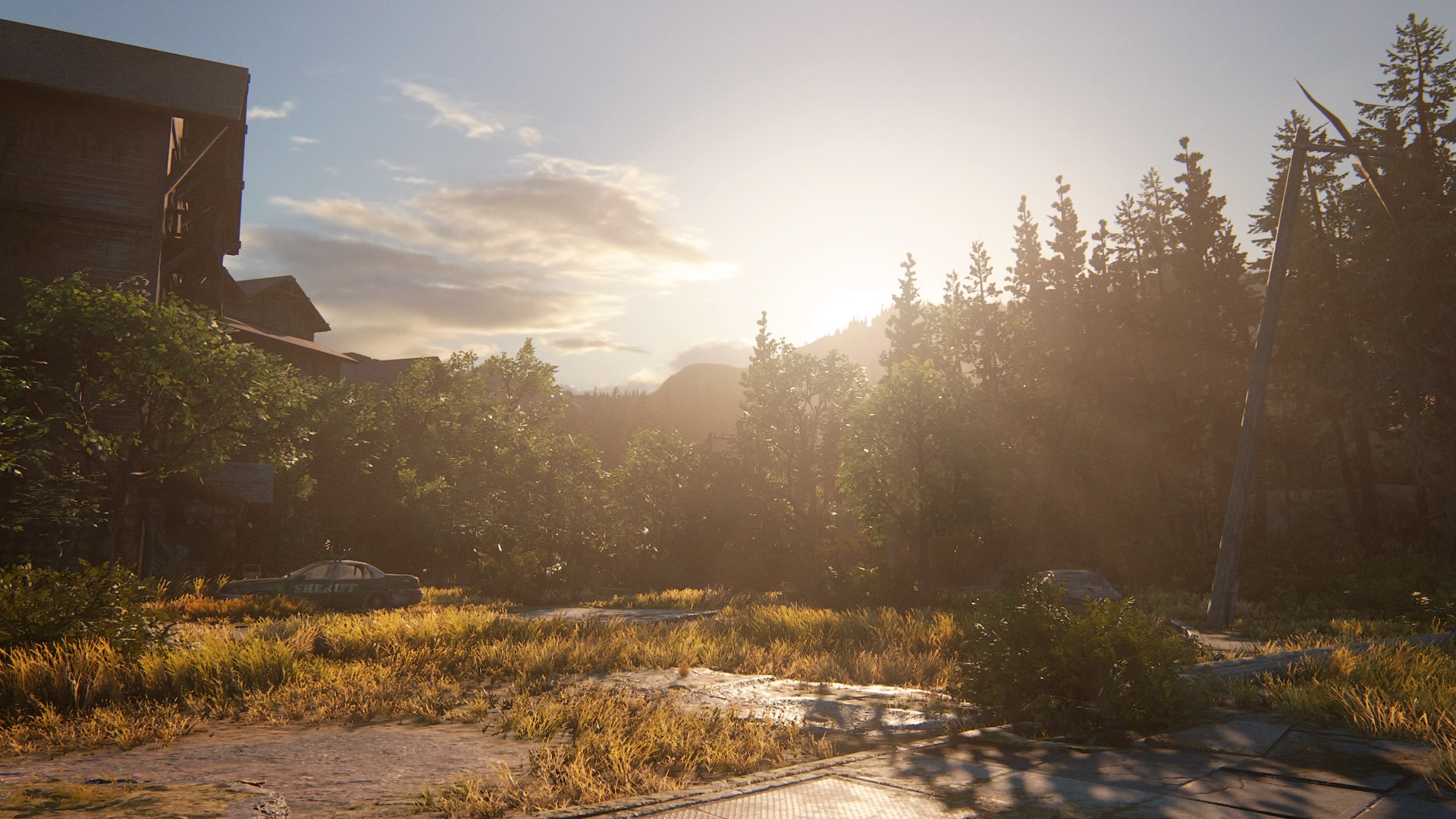The image is a screenshot from a video game or a computer-generated scene taken outdoors during the day in landscape mode. The sky is a vibrant blue, especially prominent on the left side, with a few large, fluffy white clouds and a bright sun almost at the center, casting white rays of light. In the background, extending from the upper left to the upper right, is a mix of deciduous trees with dense green leaves on the left and tall evergreen or pine trees with larger, black trunks on the right. 

On the left side, there is a multi-story building that transitions in color from gray at the top to brown as it goes down. A sheriff's car, clearly computer-generated, is parked in front of this building. It is mostly gray with barely readable text that says "sheriff" on it. Additionally, there is a tall pole towards the right of the image.

In the foreground, the ground is covered with well-maintained grass. There are also black concrete pavers overgrown with grass, suggesting a natural, somewhat untamed setting. The overall composition and the distinct, detailed textures suggest a meticulously crafted digital environment.